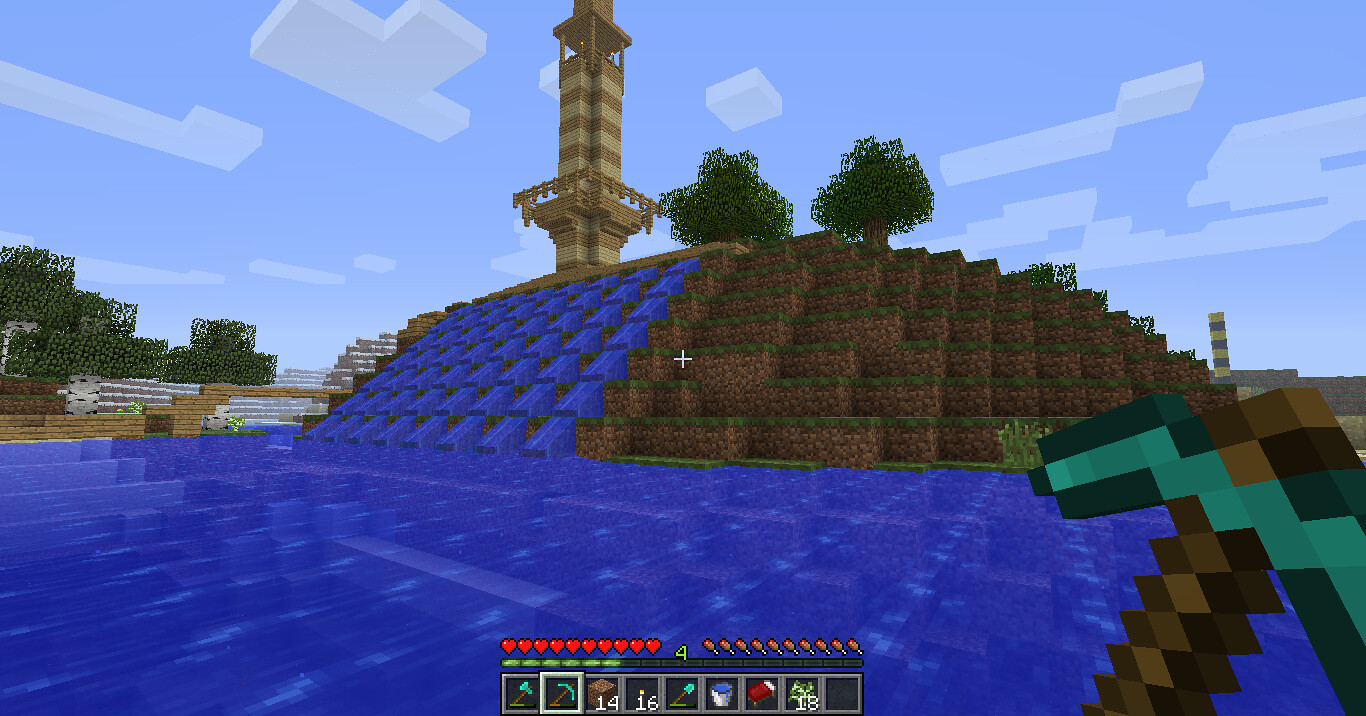The image depicts a pixelated, blocky computer game scene with a prominent focus on water. The main feature of the image is a blue body of water that ascends at an angle, giving the impression of a waterfall flowing uphill. Centrally positioned is a hill that tilts to the left. Atop the hill stand two trees alongside a tower. The tower features a small balcony at its base and extends upwards, resembling a bell tower. The overall aesthetic is characterized by retro-style pixel graphics, adding a nostalgic touch to the landscape.